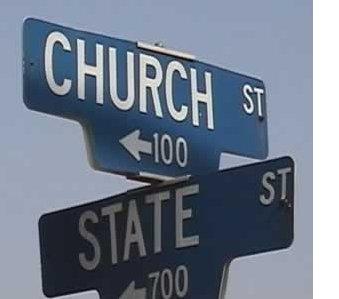This image is a color photograph taken outside, capturing a close-up view of two street signs at an intersection. The photograph, which appears to be in a slightly compressed and low-resolution format, shows some JPEG artifacting around the signs. Both signs are designed to provide direction and feature white lettering on a blue background. The top sign reads "CHURCH STREET" and includes a white arrow pointing to the top left, with the number "100" beside it. Below it, an identical sign reads "STATE STREET," displaying an arrow that points to the left, but slightly more towards the left than the arrow above, with the number "700" beside it. The vibrant, perfectly blue sky serves as the backdrop, enhancing the visual clarity of the signs despite the low resolution and minor artifacting. The image is in square format and gives an impression of realistic, potentially drone-captured photographic representation.